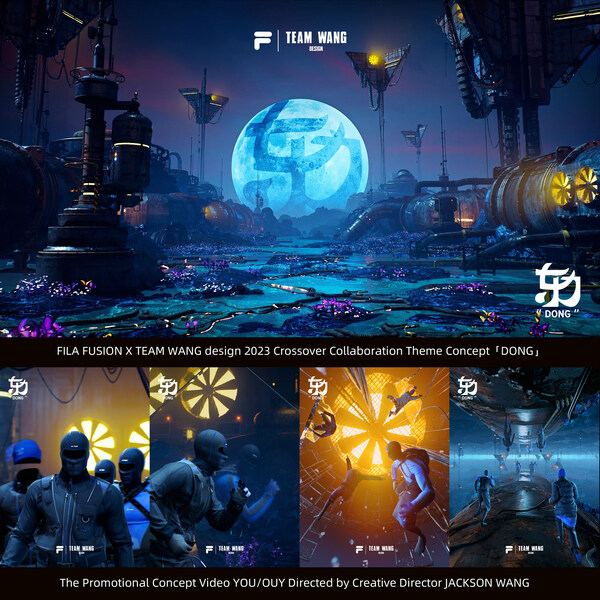This highly detailed digital image, likely created using digital animation software, showcases a futuristic, science fiction-themed scene filled with metallic, shiny objects and intricate spiral designs emitting light. The composition consists of a large upper section and a divided lower section with four smaller scenes. The top of the image features text stating "Team Wang," set against a vibrant, fantasy-like planetary surface with alien plant life and a moon with symbols, suggesting an otherworldly setting.

The central theme is accentuated by vivid blue and purple hues, enhancing the futuristic, end-of-the-world vibe. Below the main image, four smaller frames depict individuals clad in dark blue or black full-body suits and masks, interacting with advanced technology in tunnel-like environments. These individuals appear engaged in various tasks, some armed with weapons like swords, implying roles as ninjas or special operatives in high-tech scenarios. Intriguingly, one image even shows people walking on the ceiling, highlighting the extraordinary technology within this universe.

The text throughout the image includes "Fusion X Team Wang design for 2023 crossover collaboration theme concept, Dong," and "promotional concept video directed by creative director, Jackson Wang," suggesting it is an advertisement for an upcoming video game or animation series.